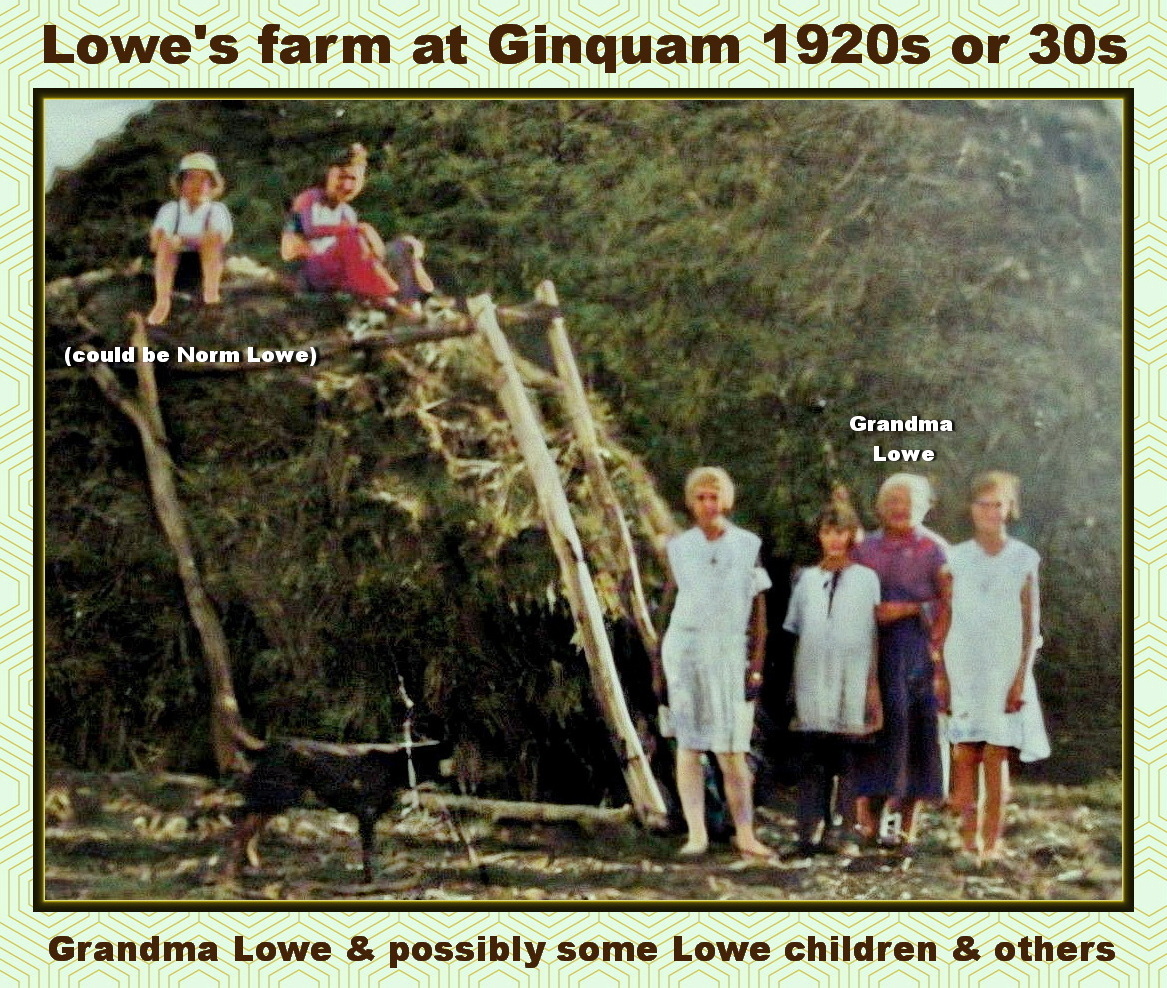The rectangular image, resembling a small poster or postcard, features a sepia-toned, old-fashioned photograph framed by a brown border. The background of the image is a light green color adorned with a pattern of concentric hexagons traced in gold. Across the top, in dark brown lettering, it reads "Lowe's Farm at Gingquam, 1920s or 30s". Similarly, at the bottom, slightly smaller brown text states, "Grandma Lowe and possibly some Lowe children and others".

The central photograph depicts a rustic farm scene with six figures, their details partially blurred. On the upper left corner, two children are seated atop a large hay bale; one child, possibly Norm Lowe, wears a cream-colored cap, white shirt with suspenders, and has bare legs, while the other child, in red pants and a striped shirt, remains unidentified. Below the children, on the ground next to the hay bale, there is a small black and cocoa-colored dog with a white splotch on its face.

To the right of the hay pile, four more figures are present. From center-right to near the image's edge, an adult woman in a sleeveless dress stands alongside a child in a white tunic shirt. Near them, an older woman, marked by the lettering "Grandma Lowe" above her head, wears a purple-pinkish top with a belt and a dark skirt. The final figure is a teenage girl in a loose, white floaty dress standing close to the photograph's edge.

The combined elements of detailed text and nostalgic imagery create a commemorative portrait of a family moment captured in time on Lowe's Farm.